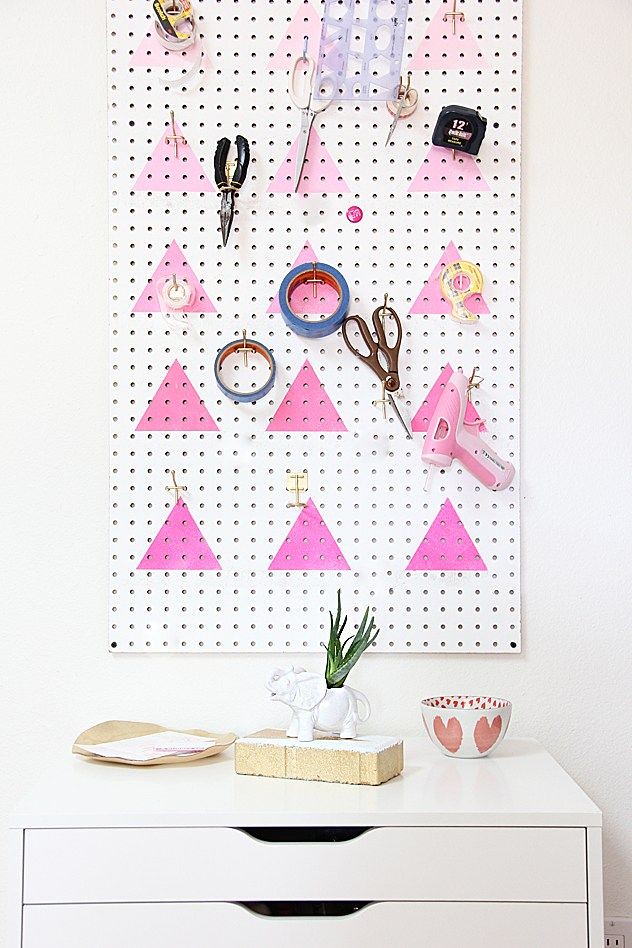In this color photograph taken indoors, we see a well-organized craft room featuring a white pegboard mounted on an off-white wall. The pegboard is decorated with pink triangles in an ombre effect, with the darkest pink at the bottom fading to lighter hues upward. Various craft tools, including scissors, pliers, a hot glue gun, painter's tape, scotch tape, and a measuring tape, are neatly hung on hooks attached to the pegboard.

Below the pegboard is the top of a white bureau with shallow drawers featuring cut-out sections for pulling them open. Atop the bureau, on the right, sits a decorative white bowl adorned with large red hearts on the outside and tiny red hearts inside. Next to the bowl, there is a painted tan brick topped with a white porcelain elephant planter. A green succulent, possibly an aloe or snake plant, emerges from the planter. To the left, a light brown tray holds a white sheet of paper. This detailed setup highlights a meticulous and artistic workspace within a cozy craft room.